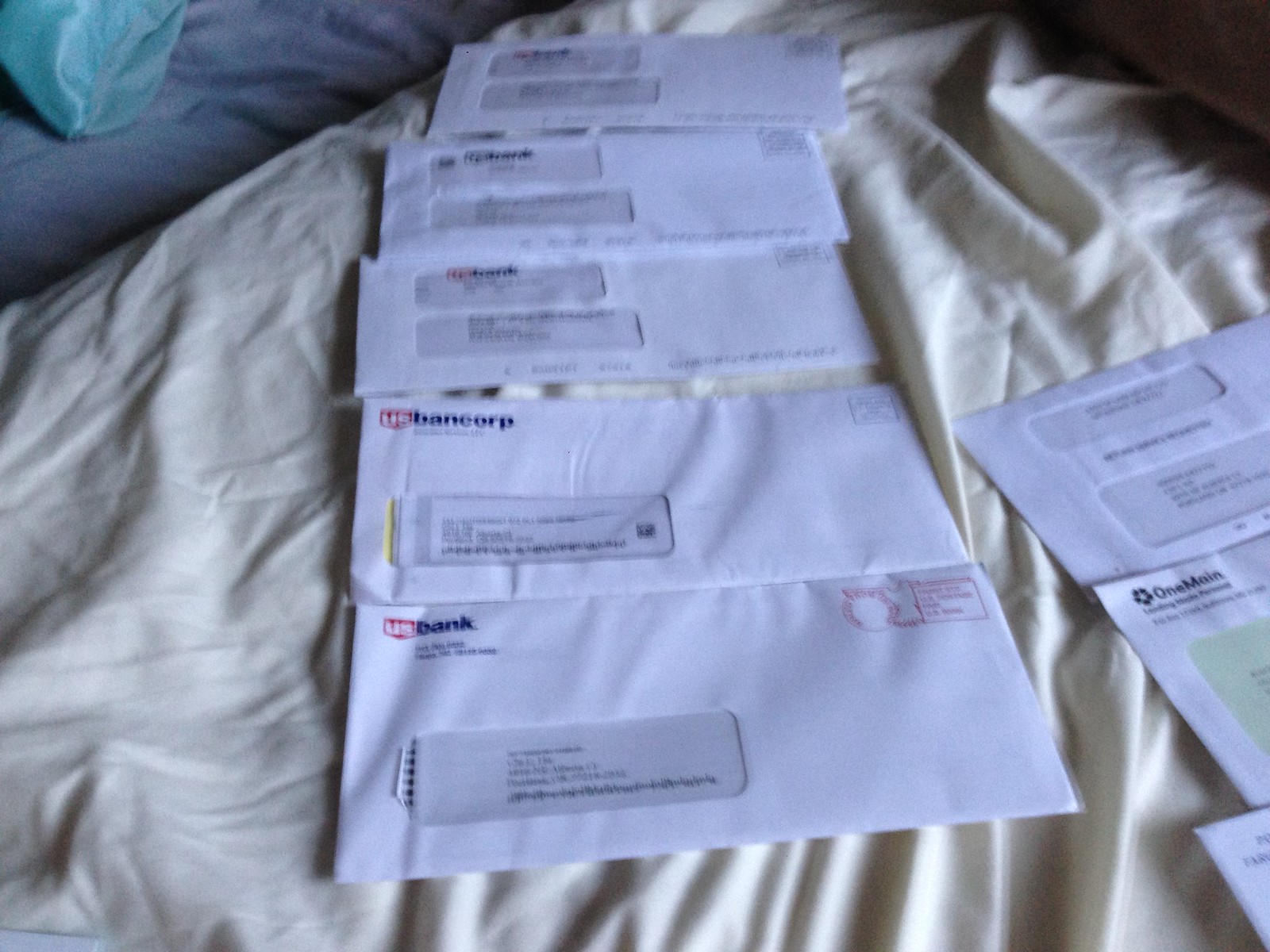This is a detailed photograph capturing various pieces of U.S. mail laid out on a bed. The bed is covered with a rumpled white sheet, and there's a glimpse of a blue sheet in the background, adding to the unmade appearance of the bed. Central in the image, there are five envelopes arranged vertically without much overlap. These envelopes mostly originate from U.S. Bank and U.S. Bancorp, identified through their glassine windows showing partial addresses. To the right of this main lineup, in the lower right corner, three more envelopes are partially visible, with one identified as being from One Main. The contents of these envelopes appear to be bills or possibly financial documents, indicated by the presence of cellophane windows revealing addresses, and none seem to be personal correspondence. The overall scene suggests that this is a close-up of someone's organized, though unkempt, display of their incoming mail and bills on their bed.